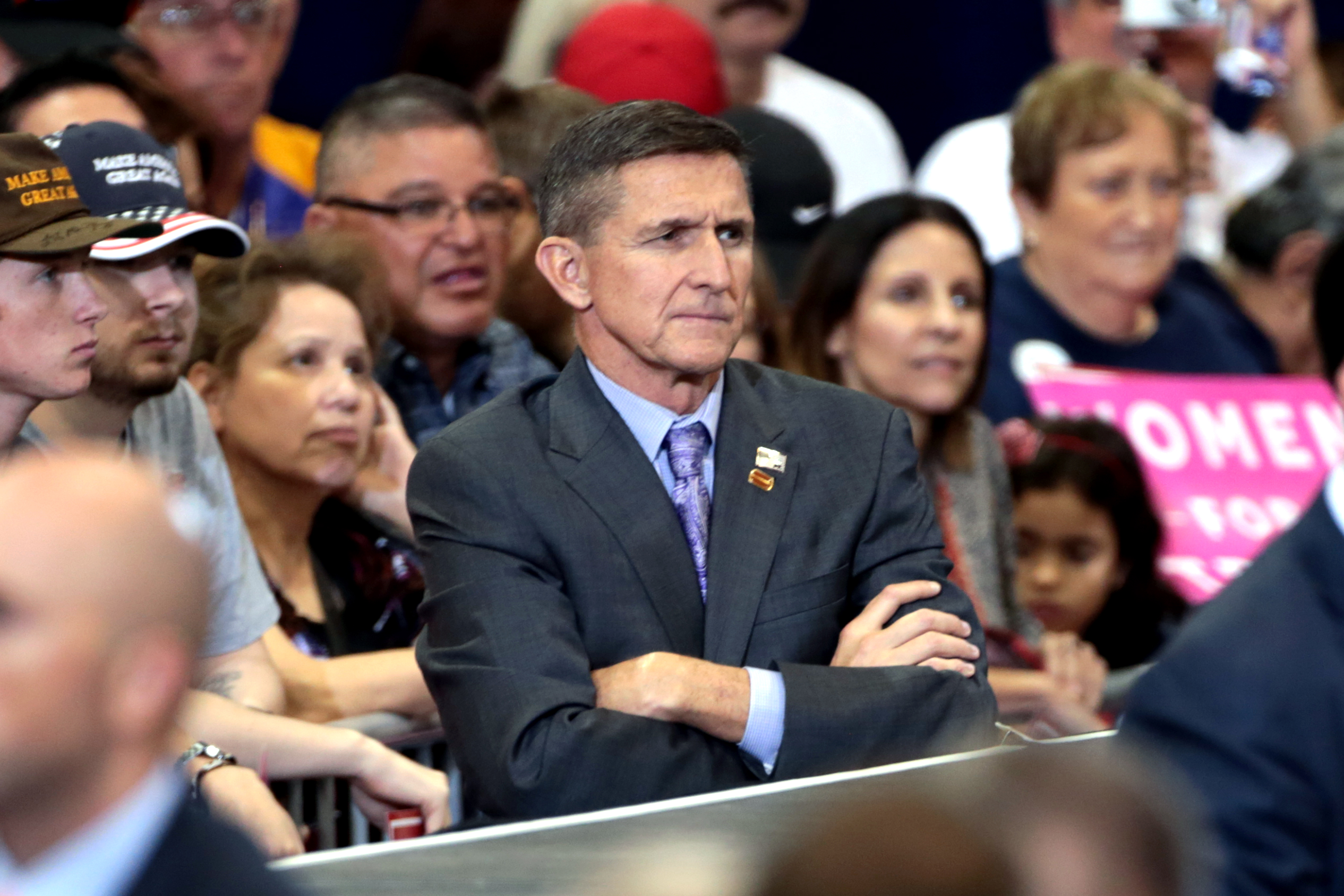The photograph depicts a distinguished, older gentleman—resembling politician Michael Flynn—standing at the front of a crowd at what appears to be a rally or public event. Flynn, estimated to be between 65 and 70 years old, is dressed in a sharp, dark blue suit adorned with pins, a light blue button-up shirt, and a coordinated blue tie. His short brown hair complements his serious, cross expression, as he stands with his arms firmly crossed. Surrounding him, a large, diverse crowd also faces the same direction, all seemingly focused on something in the distance. Behind Flynn, the crowd includes individuals of various ages, some wearing "Make America Great Again" hats, and they are gathered behind a metal or concrete barrier that separates them from him. A few indistinct figures, likely security personnel, can be seen beyond the barrier, adding to the atmosphere of controlled access and heightened security. The entire scene suggests a significant event, with Flynn standing in a prominent position, both physically and symbolically, separated from the crowd.